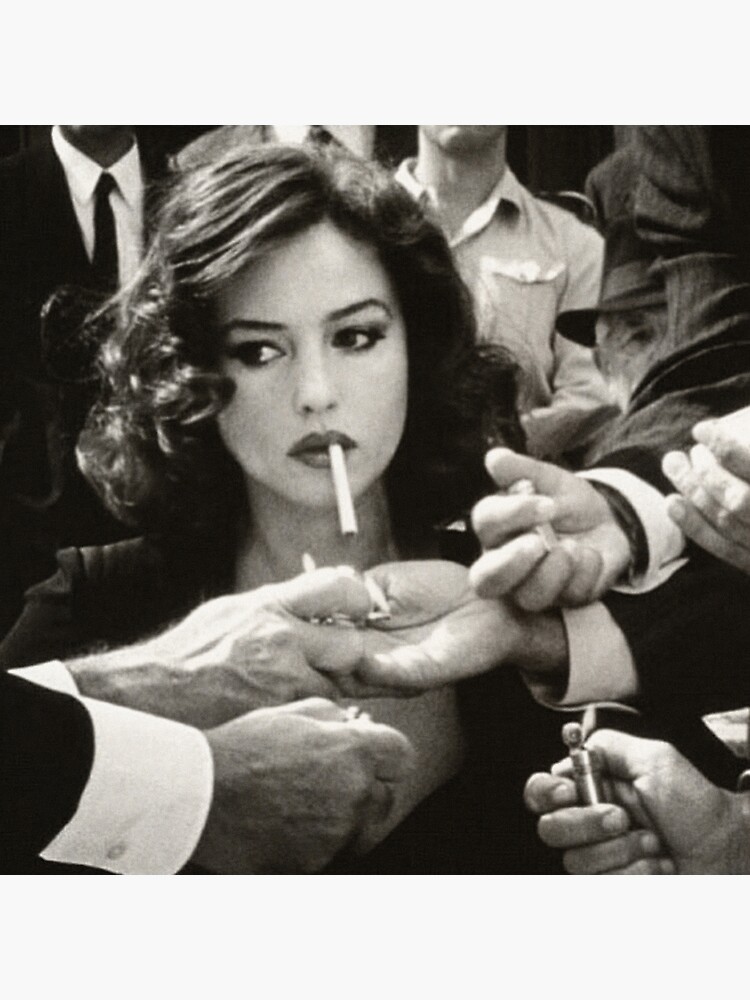In this black and white photograph, a woman with dark, curly hair and striking makeup, including red lipstick and dark eyebrows, stands in the foreground. She is wearing a low-cut dress or a stylish black jacket, exuding an air of elegance and effort in her appearance. Her head is turned slightly to the left, and she holds an unlit cigarette between her lips. Around her, at least five sets of male hands extend towards her, each holding lighters, creating a striking contrast against her poised demeanor. The background reveals several men dressed in business attire, including dark suits, white collared shirts, and even a fedora, though their faces are cropped out of the frame. The scene, reminiscent of the 1950s or 60s due to the fashion and black-and-white styling, suggests a glamorous moment possibly capturing a movie star amidst admiring gentlemen.